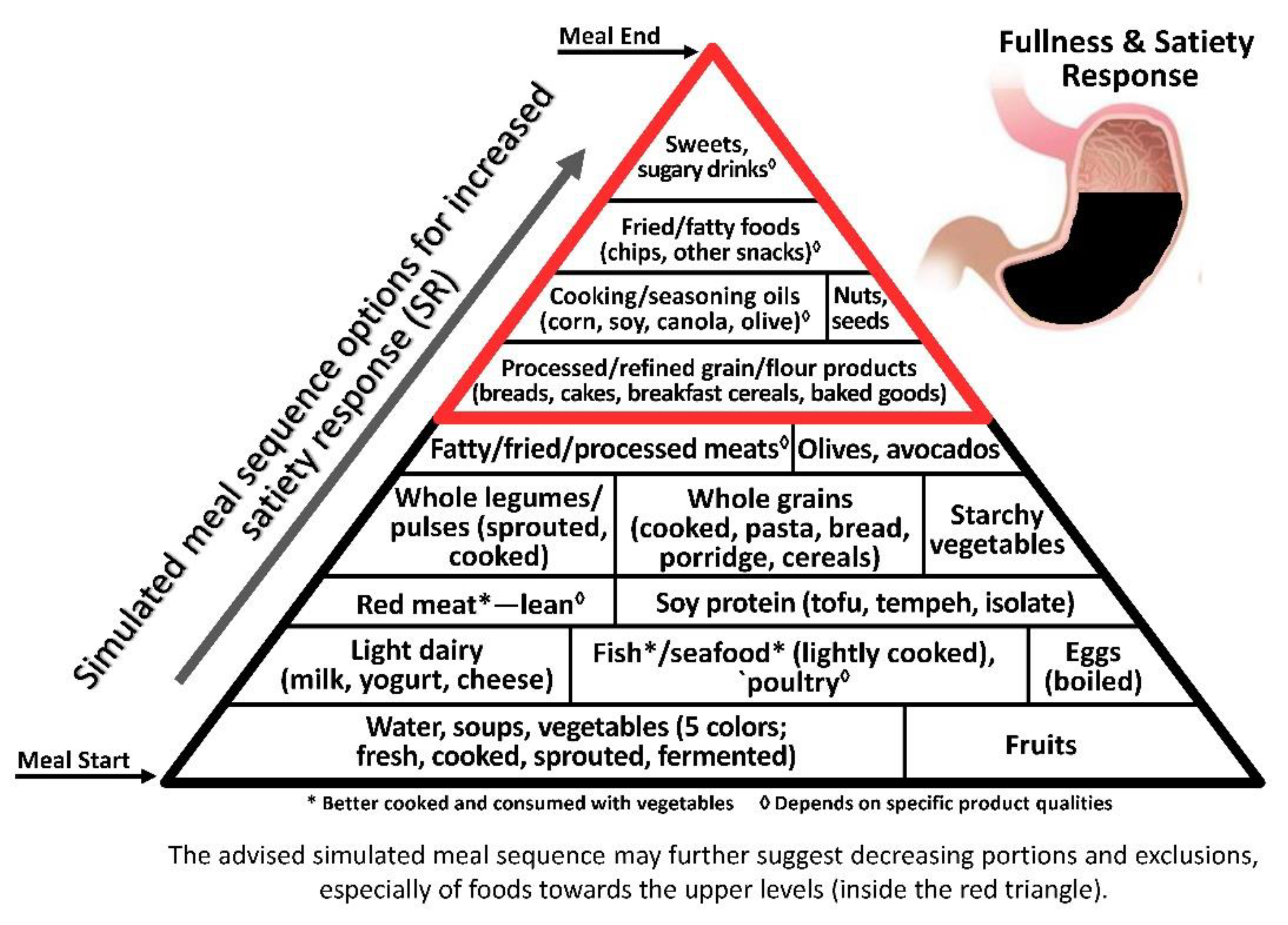The image is a pyramid diagram illustrating various food groups organized by their effect on satiety and meal sequence. The pyramid is segmented into multiple sections, with the bottom labeled as "Meal Start" and the top as "Meal End." Arrows annotate the transition from bottom to top, indicating "Simulated Meal Sequence Options for Increased Satiety Response (SR)." The bottom section is black and contains healthy options such as fried fatty meats, olives, and avocados. As you move upward, the diagram transitions to a red section containing less healthy options like sweets, fatty foods, and cooking oils. To the right of the pyramid is a detailed illustration of a stomach, depicting a pink esophagus leading into the stomach and brown intestines leading out, with a black shading inside the stomach representing fullness. Text accompanying the stomach image reads "Fullness and Satiety Response." At the base of the pyramid, additional advice suggests decreasing portions and excluding foods found in the upper segments for better health benefits.